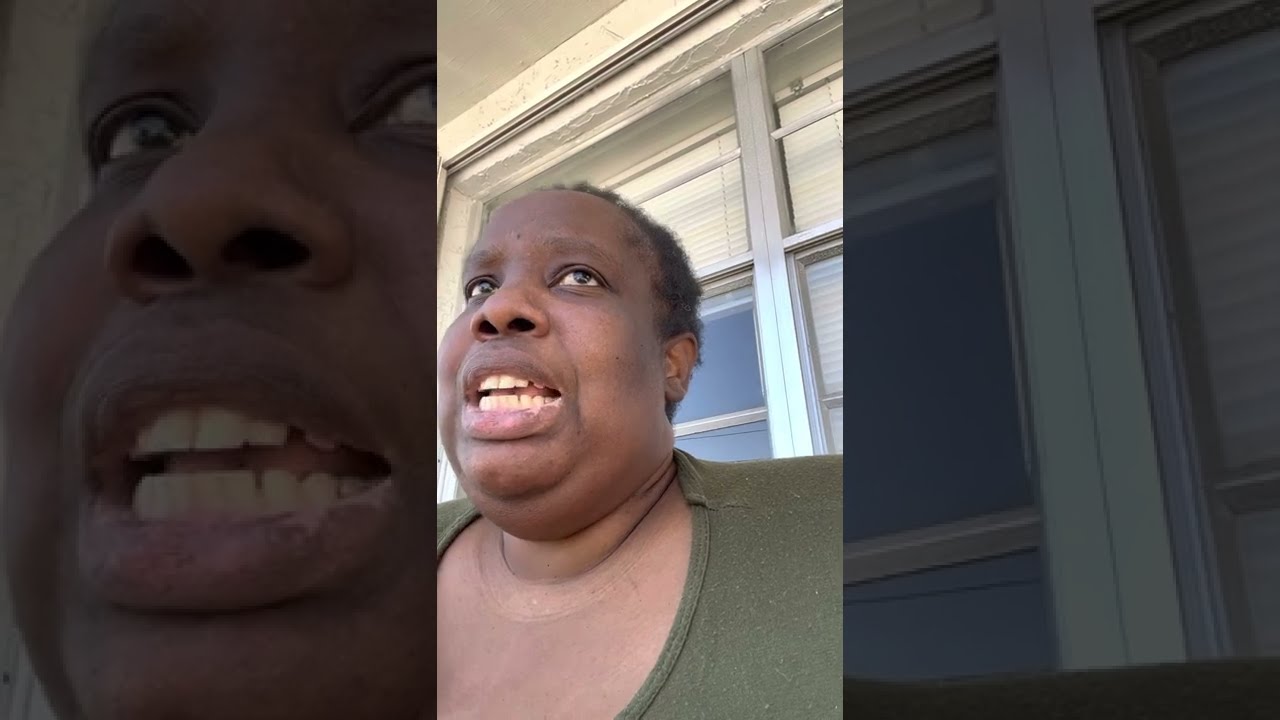The image depicts a distraught Black woman with dark brown skin, wearing a green t-shirt adorned with a circular design. Her short, raggedy hair reveals a slight receding hairline, and her black eyes are uniquely positioned—her head is slightly angled to the left while her eyes, filled with emotion, glance back to the right. Her mouth is open, revealing both her top and bottom teeth along with a bit of her tongue, and she has a noticeable double chin.

The photograph is divided into three equal vertical segments. The central segment presents a normal, bright section of the image, where the woman stands in front of a large white window framed in silver. The window blinds are down, except for a small portion directly behind her head where they are open, letting light shine through. 

The segments on the left and right are darker with a shadowy hue. The left segment features a close-up zoom of the woman's face, focusing on her open mouth, nose, and eyes, emphasizing her emotional state. The right segment zooms in on the portion of the window behind her, highlighting the details of the blinds and creating a sense of depth and continuity to the background. This triptych format emphasizes the woman's emotional expression and the setting, giving a detailed and poignant portrayal.